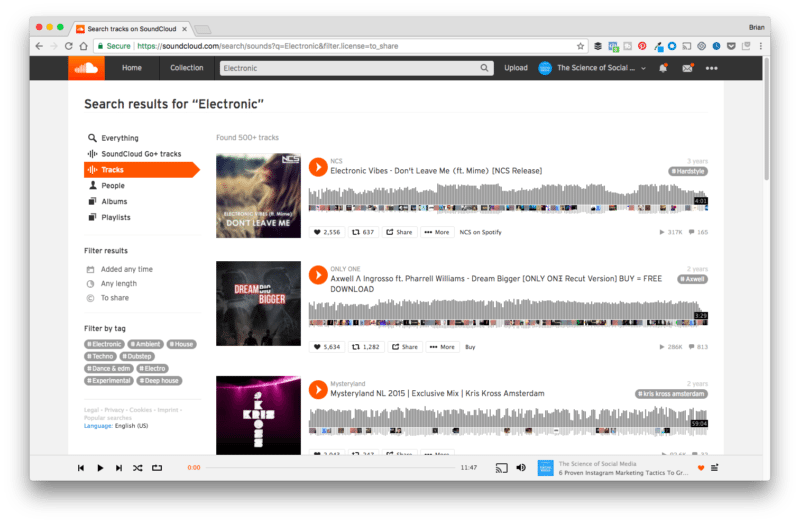This is a detailed screenshot of a SoundCloud page displayed in a web browser. At the top tab, it reads "Search tracks on SoundCloud" next to an orange square featuring a white cloud logo, signifying the SoundCloud logo. In the browser's address bar, a green text "Secure" and a green lock icon are prominently shown, indicating a secure connection. The URL following this is "https://soundcloud.com/search/sounds?q=electronic&filter.license=to_share". 

Below the address bar, the main SoundCloud webpage is visible. The top section is a black header bar with the SoundCloud logo on the left side. To the right of the logo, the menu options include "Home" and "Collection" in white text, followed by a gray search bar with the word "Electronic" typed in gray text and a gray magnifying glass icon on its right. Further to the right on the black header are the options "Upload" and a truncated "The science of social..." text. A blue profile picture with unreadable white text is next, adjacent to a white bell icon with an orange dot in its top right corner, a white envelope icon with a similar orange dot, and finally, three white dots indicating more options.

The main content area underneath this header has a white background that begins with the header "Search results for 'Electronic'" in large gray text at the top left. The search results display three items. 

1. The first result features an album cover with the image of a long-haired person standing in a wheat field with white text reading "Don't Leave Me". To the right is a gray waveform of the song labeled "Electronic Vibes – Don't Leave Me (feat. Mime) [NCS Release] #Hardstyle", with artist name "NCS" displayed above. An orange circle with a white play button in the center is also present.

2. Beneath this, the second result is titled "By Only One" by Axwell Λ Ingrosso featuring Pharrell Williams - "Dream Bigger" (Only On Recut Version) [Free Download] with a corresponding gray waveform below the description.

3. The third search result is mentioned but not described in detail.

This screenshot captures the detailed interface and current search results for "Electronic" on SoundCloud, highlighting the visual and interactive elements of the platform.